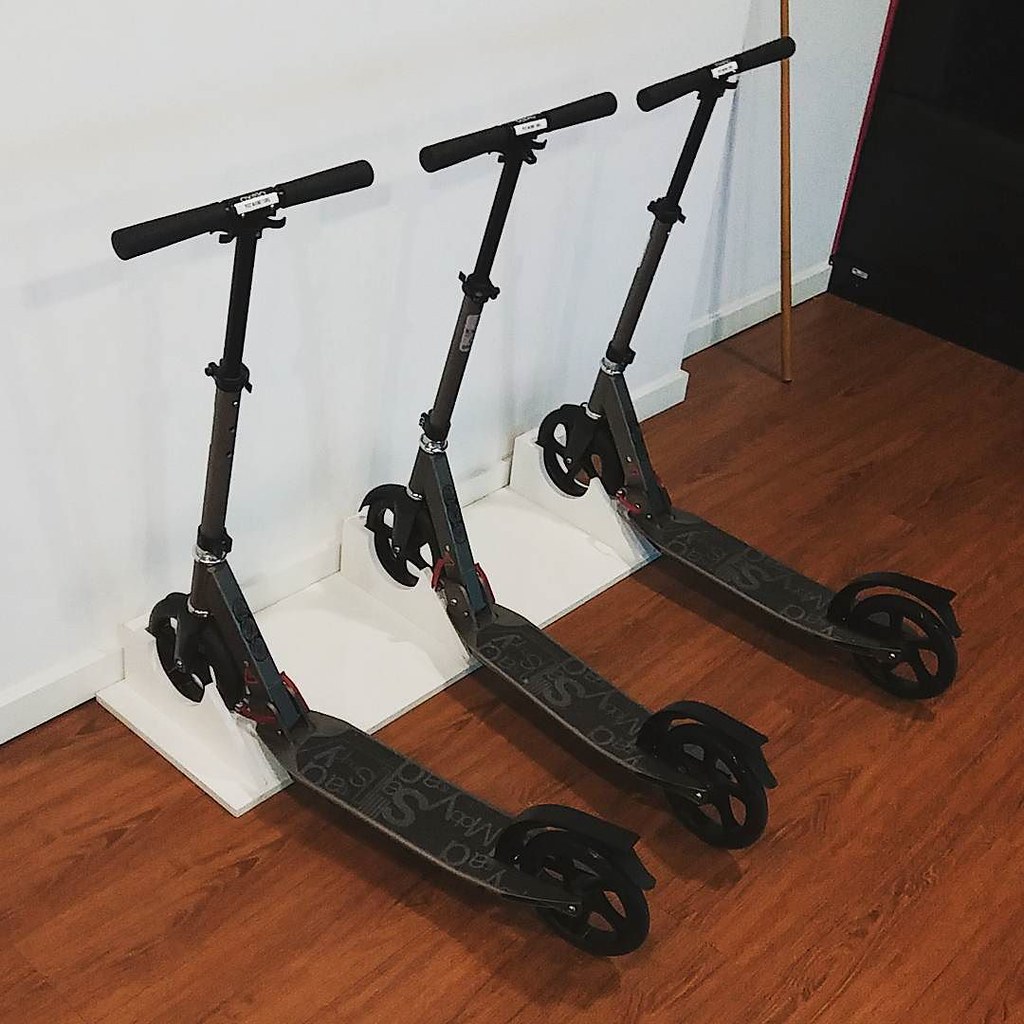The image depicts an indoor scene featuring a white-painted wall and a medium-rich or bright brown wooden floor. Against the white wall, there is a white square docking station, designed to hold scooters. The docking station features three slots, each occupied by a black scooter. All the scooters are identical in appearance; they have black wheels, black handlebars, and a black baseboard with some sort of matte colored lettering, although the exact text is indiscernible. The floor is oriented at an angle, extending from the bottom left to the upper right of the photograph. Additionally, in the upper right corner, there appears to be a wooden pole standing against the wall, and possibly a door or another object nearby.